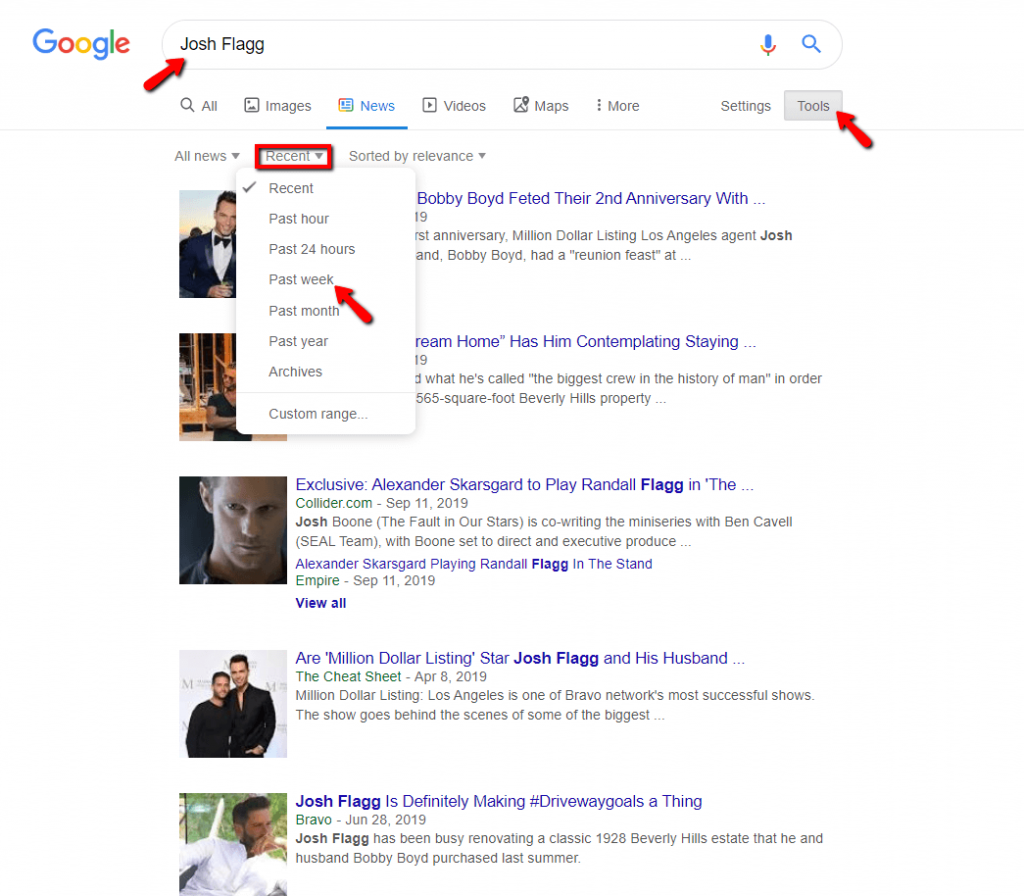**Detailed Caption**:

The image is a detailed screenshot of a Google search news results page. Starting from the top left, the vibrant Google logo is displayed in its signature colors: a blue "G," followed by a red "O," a yellow "O," a blue "G," a green "L," and a red "E." To the right of the logo, a search bar shows the query entered by the user: "Josh Flagg." Highlighted by a red arrow with a shadow effect pointing directly at the text, the search bar also contains the microphone icon and a blue search button to its right.

Below the search bar is the tabs section allowing the user to switch between different search result categories. The tabs read: "All," "Images," "News," highlighted in blue with a blue underline, "Videos," "Maps," and "More," marked by a three-dot icon. To the right of these tabs are options for "Settings" and a button labeled "Tools" inside a gray box, accentuated by another red arrow pointing at it.

A thin gray line separates the tab section from the filters section below. The first row includes "All News" with a drop-down arrow, and "Recent," also with a drop-down arrow. In this row, there is an expanded drop-down menu showcased by the user's additional editing, which includes a red rectangle around "Recent." The drop-down menu reveals selection options for filtering news results: "Recent" (checked), "Past hour," "Past 24 hours," "Past week" (highlighted by a red arrow), "Past month," "Past year," "Archives," and "Custom range." To the right of these options is "Sorted by relevance."

The drop-down menu partially obstructs the visible search results beneath it. The first visible news result reveals a thumbnail image on the left, depicting Josh Flagg in a tuxedo. To the right, part of the text reads, "Bobby Boyd feted their second anniversary with..." and concludes on the next line with "anniversary million-dollar listing Los Angeles, agent Josh..." followed by the continuation in which, "and Bobby Boyd had a reunion feast at..." The subsequent news item follows a similar layout: a thumbnail image to the left with the obscured title and some subtext below it. The third, fourth, and fifth results follow the same format, albeit partially obscured by the drop-down menu.

This extensively detailed image reflects a thorough search query about Josh Flagg within Google news results and highlights specific user-driven edits to accentuate certain elements on the screen.